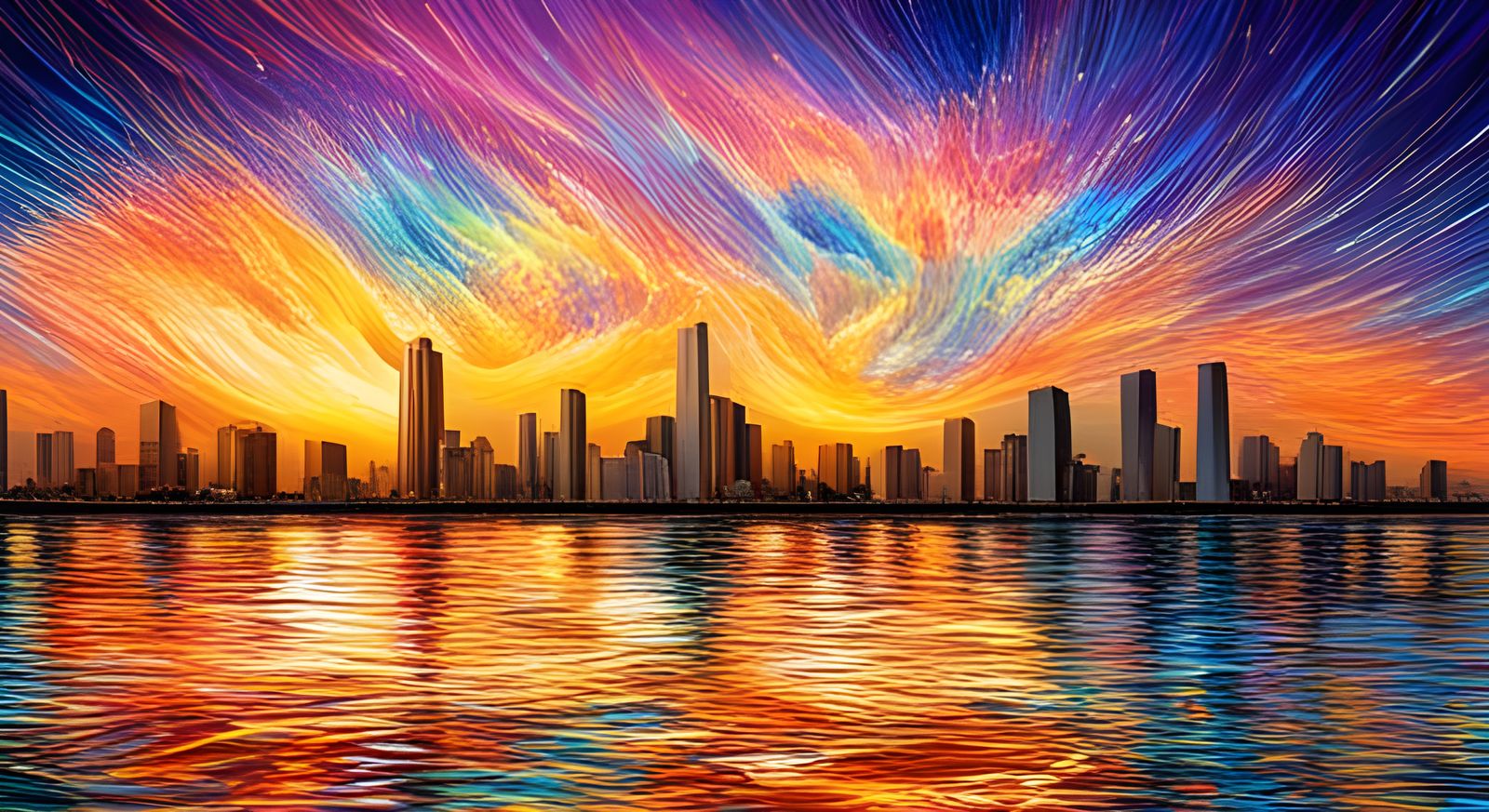The image is a highly detailed, computer-generated illustration of a modern city skyline at night, viewed from a body of water. The urban landscape, with its towering buildings, is positioned centrally in the composition. Surrounding the city's edge is a lake or sea with slightly choppy waters that mirror the vibrant colors of the sky above. The sky itself is a stunning artistic representation, dominated by swirling hues of red, orange, gold, purple, and some blue and pink. These colors form an aura-like display reminiscent of the Northern Lights, creating a dynamic, almost time-lapsed effect with streaks of light extending from the bottom to the top of the image. The reflective and glistening quality of the water enhances the mesmerizing effect of the sky's colors, making the entire scene appear both magical and vividly lifelike.